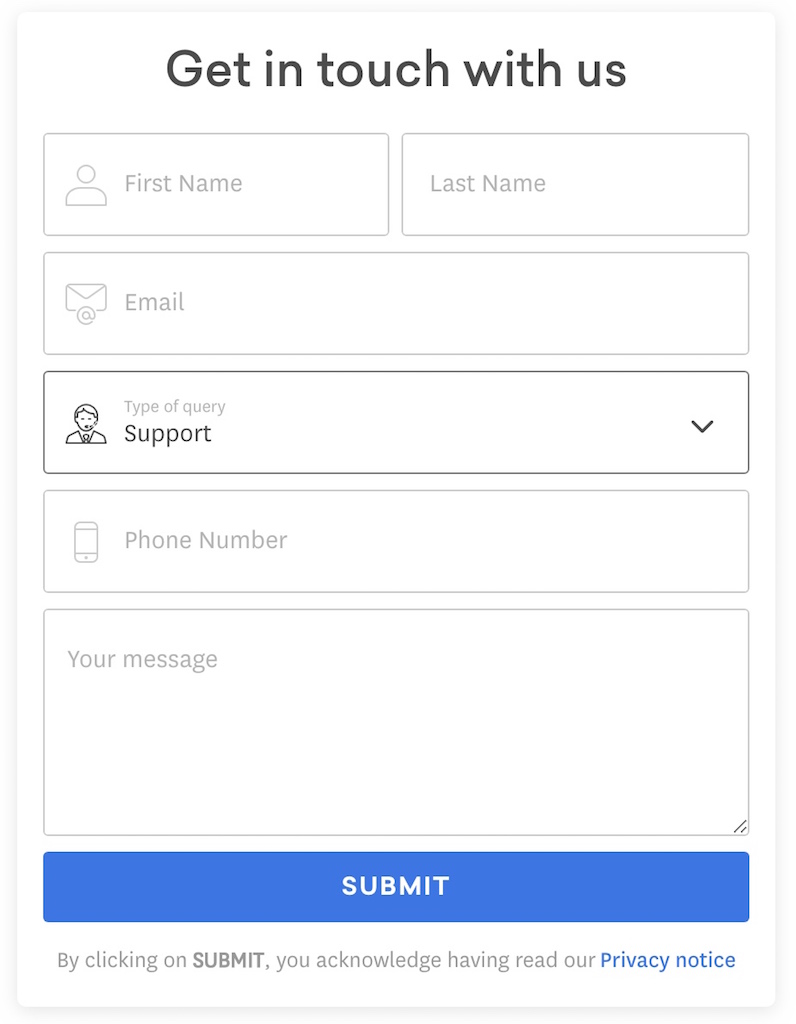This is a screenshot of a "Get In Touch With Us" screen, which appears to be displayed on either a mobile device or a computer. At the very top of the screen, there is a bold header that reads, "Get In Touch With Us." Below the header, there are various input fields arranged vertically for user interaction. 

The first field is a text box labeled "First Name," followed by another text box labeled "Last Name." Underneath the name fields, there is a text box for "Email," which collects the user's email address. 

Next, there is a dropdown menu labeled "Type of Query," with the currently selected option being "Support." Further down, there is a text box for "Phone Number," allowing users to input their contact number. Below the phone number field is a larger text area where users can type their detailed message or inquiry. 

At the very bottom of the screen, there is a prominent blue "Submit" button, which users can click to send their information and message.